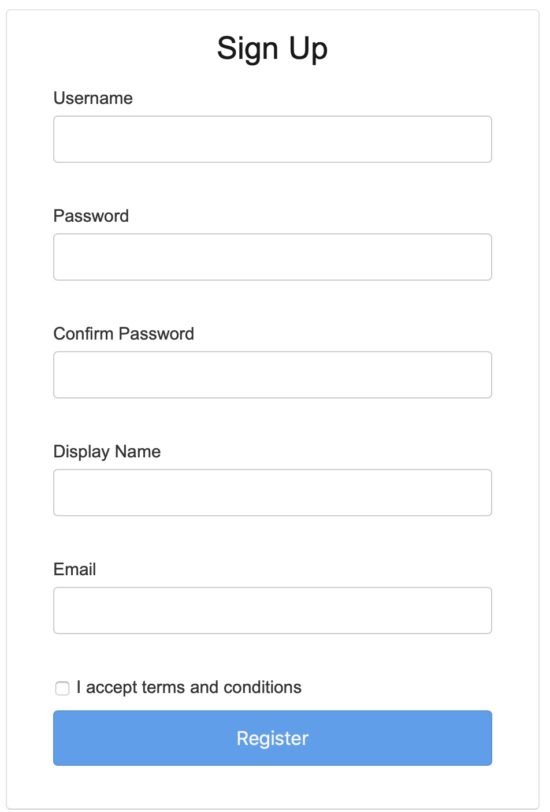A minimalist registration form on a website is depicted with a purely white background. At the top of the form, "Sign Up" is prominently displayed in black letters. Below, "Username" is indicated in smaller black text, accompanied by an empty input box for the user to enter their username. The form proceeds to request a "Password" directly underneath, with a corresponding empty input box for the user to fill in their desired password. Directly below, a "Confirm Password" field follows the same format, requiring the user to re-enter their password. Next, there is a "Display Name" label with an empty input box for the user's chosen display name, and subsequently, an "Email" label with an input box for the user's email address. Additionally, a small checkbox is present with the text "I accept terms and conditions" adjacent to it, indicating that the user must accept the terms before proceeding. At the bottom of the form, a distinct blue button with "Register" inscribed in white letters stands out, ready to finalize the sign-up process upon completion of the required fields. All textual elements are in black, contributing to the clear and straightforward presentation of the registration form. The form is standard and unfilled, offering no personal details or specific information about the type of website it belongs to, implying it is a generic example of a common web form. The terms and conditions mentioned are not visible within the form.